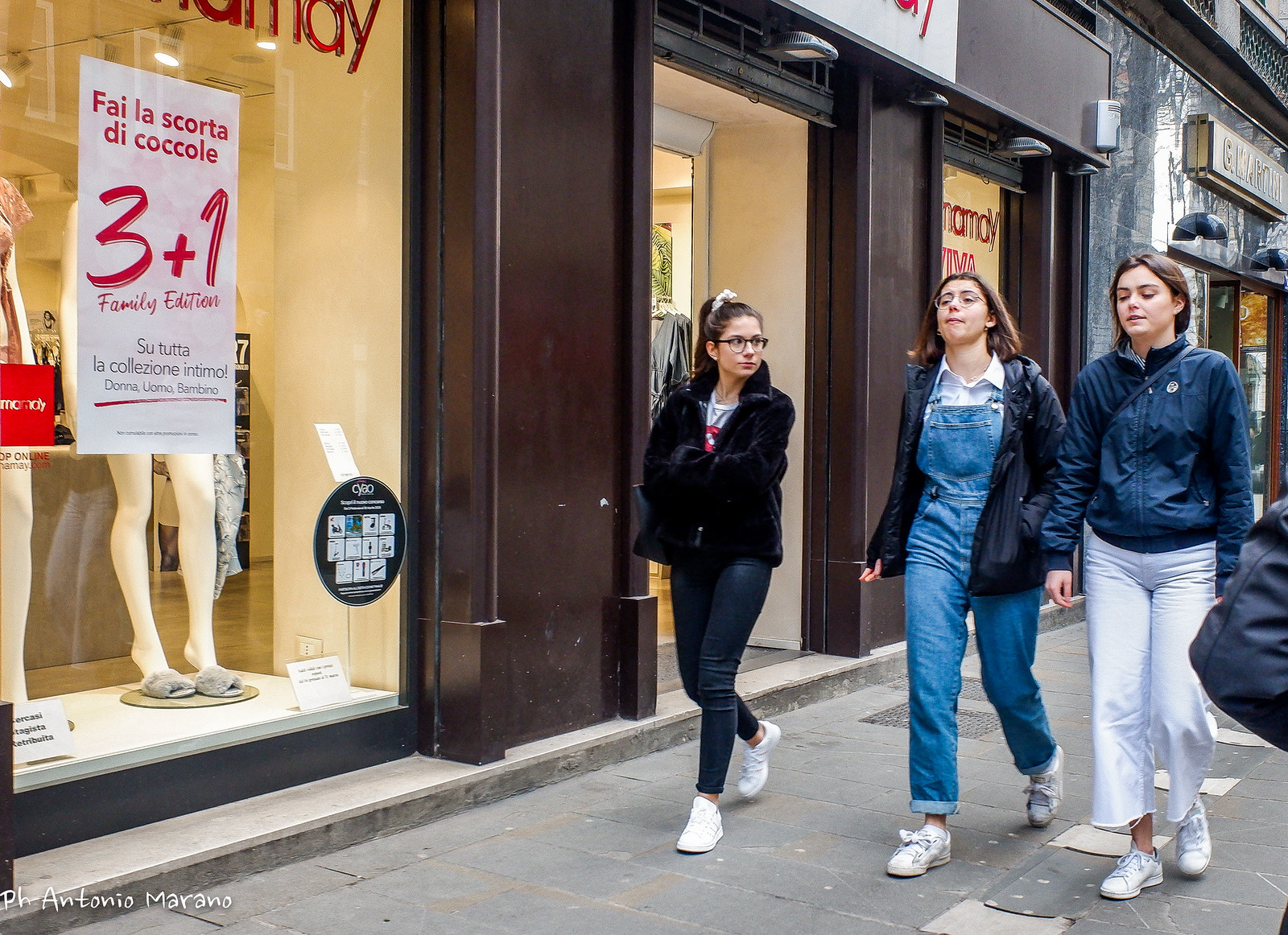This photograph captures three young women, likely teenagers or in their early twenties, walking side by side on a city sidewalk near various storefronts. The scene is likely set in a Spanish or Portuguese-speaking country, as indicated by the signs in the background. The sidewalk is composed of gray rectangular bricks, and the buildings are dark brown with large windows. 

To the left of the frame is a sizable window with a partially visible sign reading "Fela Scorta D coso cocoa CEO CEO le." Another noticeable sign in the window is a white advertisement with the words "3 plus 1 family edition" in red letters, hinting that they are passing by a clothing store with mannequins visible in the display.

The young woman on the left is dressed in a black fuzzy jacket, black leggings, and white tennis shoes. She has her hair pulled up in a ponytail with a white scrunchie and is wearing eyeglasses. She appears to be giving a side glance to the others.

In the center, another woman sports a denim jumpsuit with a black jacket over it. She has straight, shoulder-length brown hair, wears glasses, and her jeans are cuffed at the hems. She also wears white tennis shoes and has a somewhat smug expression as she looks straight ahead.

The third woman, on the right, is clad in a blue jacket and white tennis shoes. She has long brown hair pulled back behind her and is wearing light blue jeans with ripped hems. She seems to be looking down as she walks along with the other two, possibly engaged in a conversation with them.

Overall, the image captures a candid moment of youthful interaction amidst an urban backdrop.